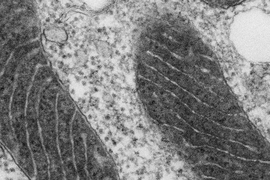In this detailed black and white photograph, which appears to be taken through a high-magnification microscope, we observe an intricate close-up of cellular structures. Dominating the panoramic-style image are two dark, peanut or lima bean-shaped forms extending vertically. These structures are textured with squiggly lines reminiscent of fingerprints, characterized by mottled dark gray patches and fine, white stripes. Between these major forms, the background is filled with a blend of light gray and black dots, creating a complex, almost abstract backdrop. In the upper right, a large white circle with a light gray squiggly border stands out, accompanied by a partial view of another similar white shape. The image altogether evokes thoughts of electron microscopy, illustrating the minute and detailed architecture of biological entities at a cellular level.